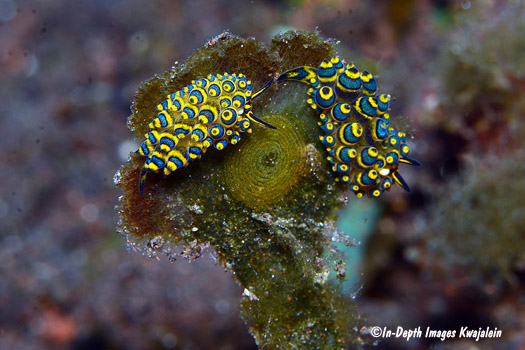The image is a close-up, underwater photograph capturing two vibrant sea slugs perched on a moss-covered, green stalk that resembles a piece of coral. Both sea slugs have cone-like structures adorned with concentric rings of bright blue and yellow. Their antennae, also blue and yellow, are prominently visible. Despite slight color variations, with the slug on the left being more yellow and the one on the right more blue, both exhibit intricate patterns of blue and yellow stripes across their bodies. The background is an out-of-focus blur blending shades of brown, burgundy, green, and red, adding depth to the image. A copyright mark, “© In-Depth Images, Kwajalein,” is positioned in the lower right corner.